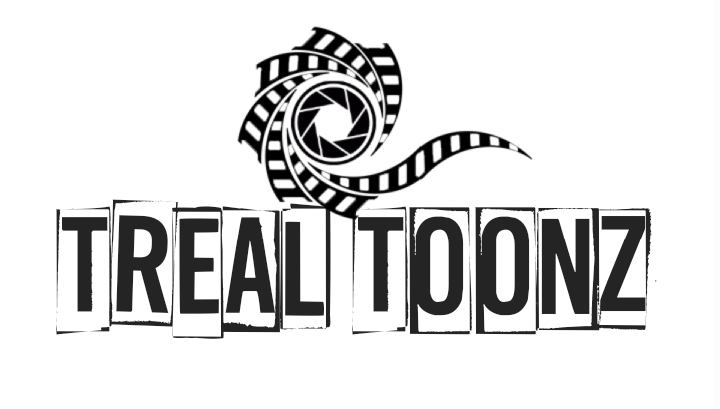The image features the logo for Trio Tunes, a music-related entity, possibly associated with sound recording or amplification. The logo is rendered in black and white. At the top of the logo, there is an intricate design resembling a swirling pinwheel or old-fashioned film reel, possibly indicative of a record spinning or film on a projector. Below this motif, the text "TRIO TUNES" is spelled out in capital letters, with each letter encased in its own square, reminiscent of cutouts from a newspaper or magazine. The overall layout of the image is upright and rectangular, with the text aligned horizontally in the center.